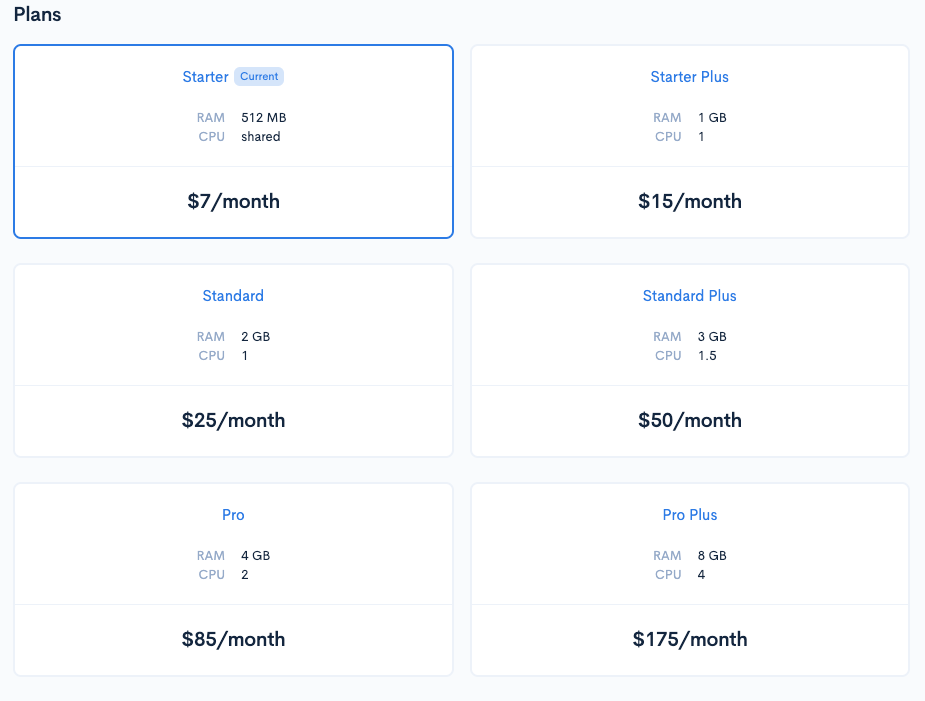This image displays a pricing chart for different monthly subscription plans, arranged within six rectangular boxes. The layout consists of two vertical columns with three rectangles each, and the title "Plans" is prominently displayed at the top in black print.

- The first rectangle on the upper left is highlighted with a darker blue border, indicating it has been selected or hovered over. This box is labeled "Starter" and details the following specifications:
  - RAM: 512MB
  - CPU: Shared
  - Price: $7 per month

- To its right, the first rectangle in the upper right column is labeled "Starter Plus" with the following features:
  - RAM: 1GB
  - CPU: 1 Core
  - Price: $15 per month

- The second rectangle in the left column is labeled "Standard," providing:
  - RAM: 2GB
  - CPU: 1 Core
  - Price: $25 per month

- Beside it, in the middle of the right column, the rectangle titled "Standard Plus" includes:
  - RAM: 3GB
  - CPU: 1.5 Cores
  - Price: $50 per month

- The bottom rectangle on the left side is marked "Pro," featuring:
  - RAM: 4GB
  - CPU: 2 Cores
  - Price: $85 per month

- Finally, the bottom rectangle on the right column is designated "Pro Plus" and shows these specifications:
  - RAM: 8GB
  - CPU: 4 Cores
  - Price: $175 per month

Each plan is distinctly outlined, providing clear information on the RAM, CPU, and cost associated with that particular selection.